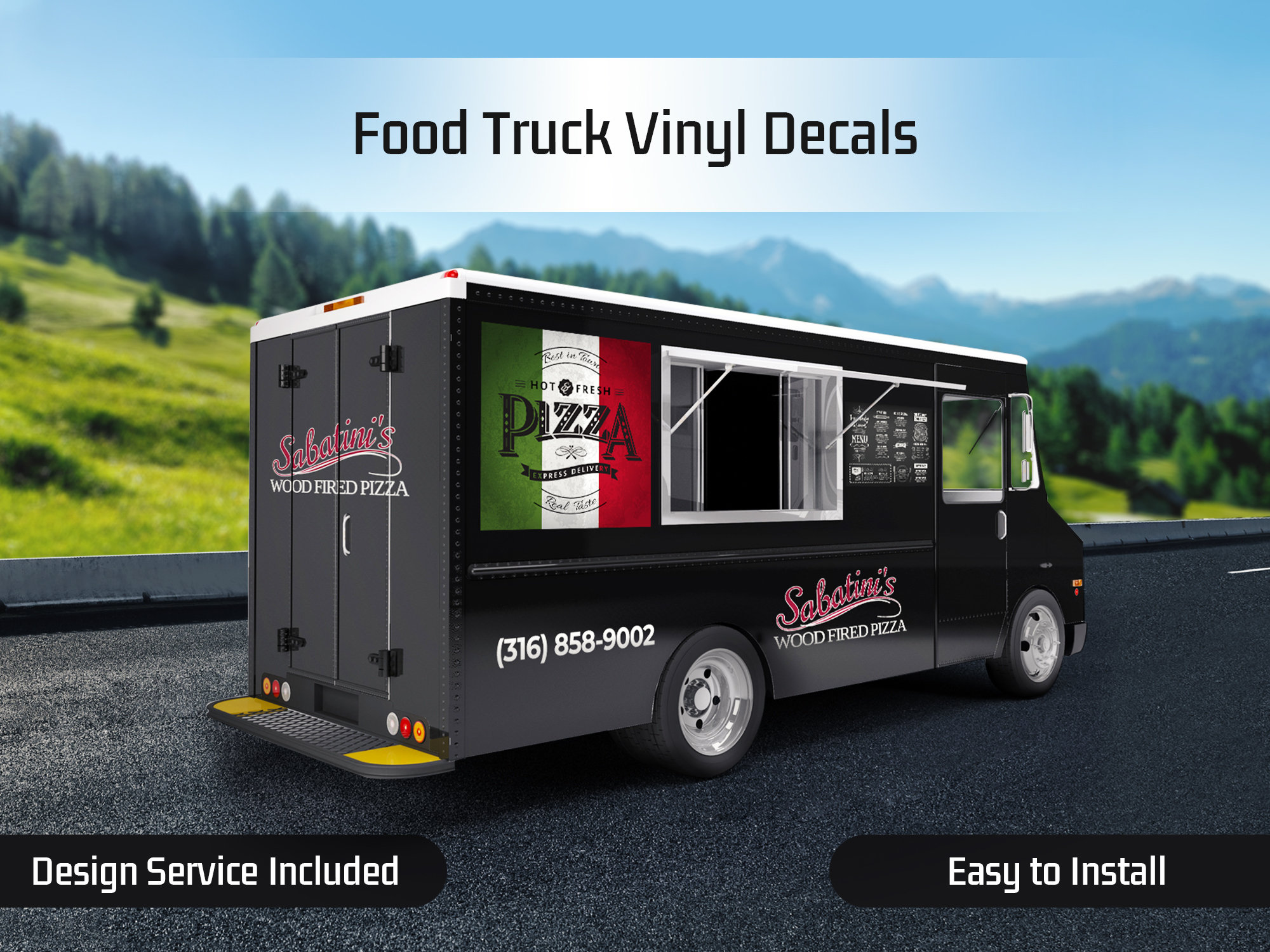The advertisement showcases a computer-generated image of a sleek black food truck adorned with various vinyl decals. At the top of the image, a white bar that thickens in the middle presents the title "Food Truck Vinyl Decals" against a blue sky. The food truck, primarily black, prominently displays "Hot and Fresh Pizza" on its side along with "Sabatini's Wood Fired Pizza" and a phone number: [316-858-9002]. A colorful emblem featuring the green, white, and red Italian flag is visible near the truck’s window. The bottom left corner of the advertisement highlights "Design Service Included," while the bottom right corner declares "Easy to Install," both set against black bars with white text. The truck, fitted with a step at the back, stands on a black asphalt road against the backdrop of rolling hills and mountains, enhancing the digitally generated aesthetic of the image.